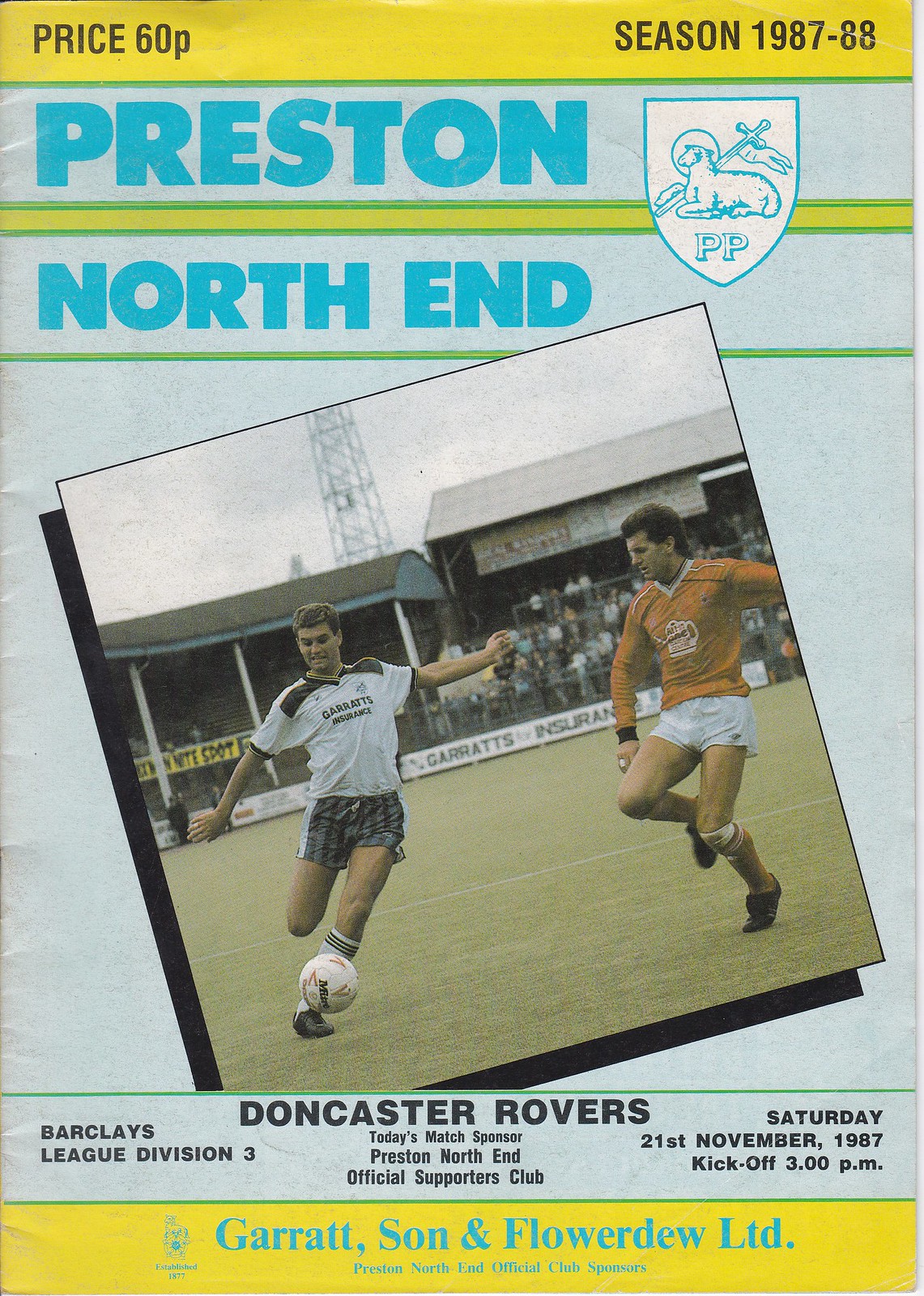This image is a detailed advertisement poster, likely the cover of a magazine, from the season 1987-88. The poster features thick yellow borders at the top and bottom. At the top, in black text, it states "Price 60p" on the left and "Season 1987-88" on the right. Below this, there is a thin horizontal green stripe followed by a light blue banner with deep blue text that reads "Preston." To the right of this text, there is a white shield with a blue outline featuring a lamb holding a cross and a banner with "P.P." written below it. This is followed by another thin yellow band and a subsequent thin green stripe.

Dominating the center of the poster is a diagonal, square photograph of a soccer match. In the image, a player in a white shirt and gray striped shorts is about to kick a ball while another player in an orange long-sleeve shirt and white shorts attempts to block him. Below this image, large black text reads "Doncaster Rovers," and to the left it says "Barclays League Division III." Beneath this, in smaller text, it states "Preston North End Official Supporters Club and Teddy's Match Sponsor." To the right, it provides match details: "Saturday, 21st November 1987, kickoff 3 p.m."

The background of the poster is a very light turquoise blue. At the bottom, within the yellow footer, blue text states "Garrett Sun, LG, LTD" with additional, hard-to-read text in smaller blue print.